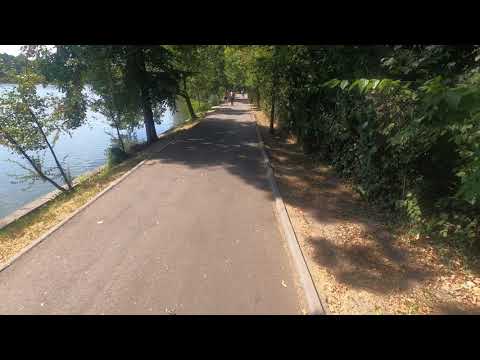The image depicts a sunlit trail flanked by natural features and vegetation. To the left, a gently sloping hill hosts a tranquil body of water, surrounded by small trees emerging from its banks. The right side of the trail is bordered by a dirt area with bushes and shrubs, offering a mix of sunlit and shaded spots, the latter provided by the trees on the left. This color image—ranging from gray to brown to blue and green—captures a daytime scene with ample natural light, suggesting clear weather. In the distance, a few indistinct figures can be seen walking along the narrow path, which resembles a walking, dog walking, or biking trail rather than a vehicle road. The path is framed by low curbs on both sides and extends towards the image's top, partially obscured by tree shade and the trail's natural bends. Overall, the scene is serene and invites a sense of outdoor recreation.